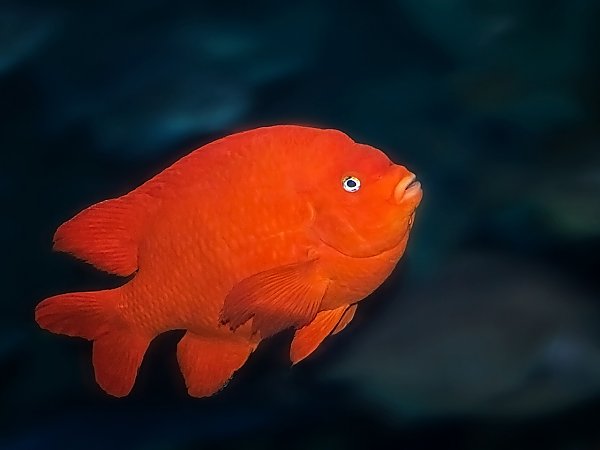The photograph features a bright, vibrantly orange fish, centrally positioned, swimming diagonally upwards towards the top right corner of the image. The fish has a distinctive silver and black eye that stands out prominently against its orange body. Its thick, light pink lips give it a slightly humorous appearance. The fish has clearly defined fins, with two sticking down, one sticking up, and a visible tail. The scales on its body run from right to left. The background is a dark, almost black hazy water, intentionally blurred by the photographer to emphasize the fish. There are no other elements, animals, or structures in the image. The scene is entirely focused on the solitary, vividly colored fish.